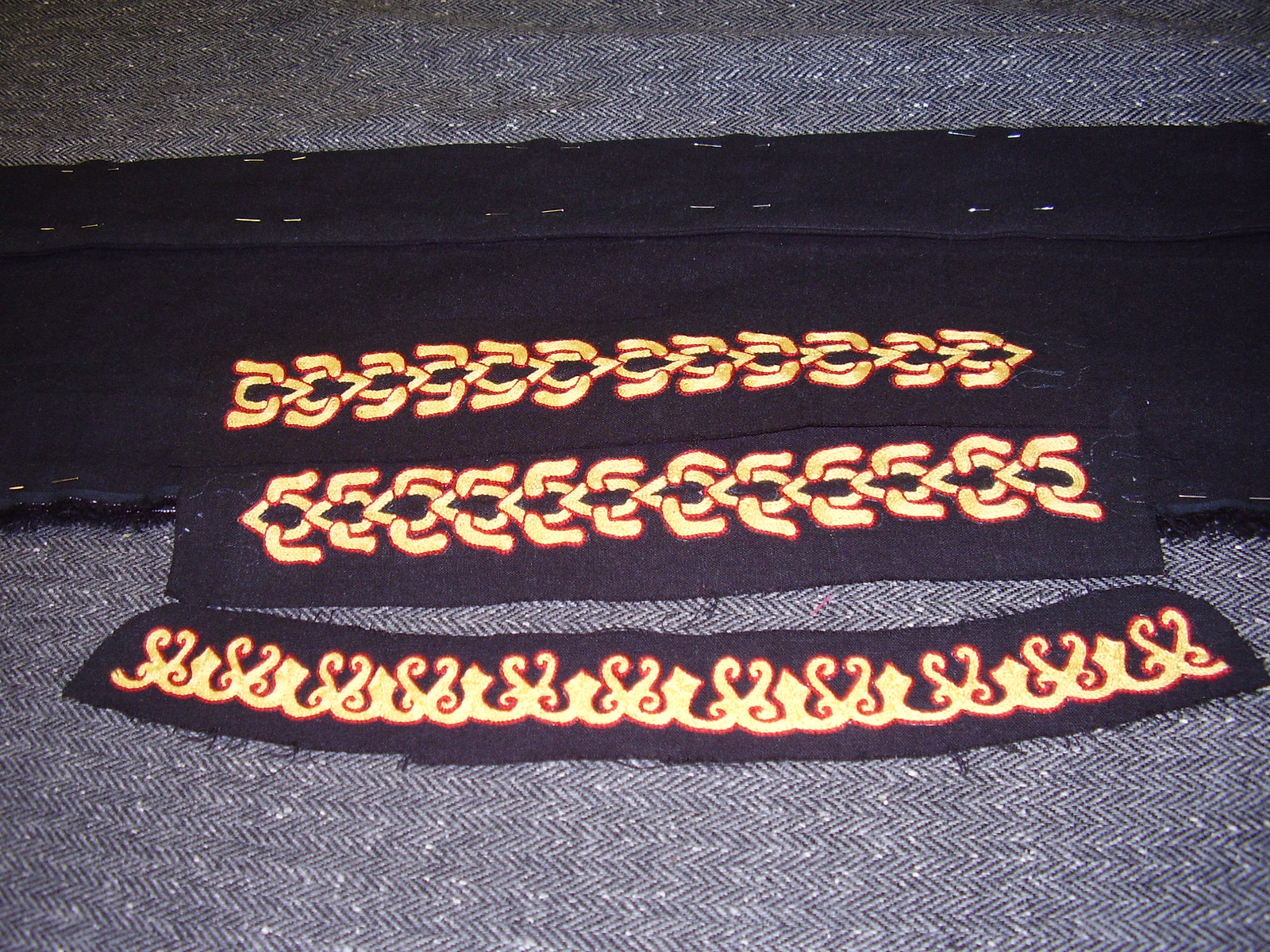The photograph features a detailed scene of sewing preparation with various components. At the base, a blue and white herringbone fabric is laid out, anchoring the entire composition. Overlaying this base, a piece of dark blue denim fabric contains meticulously folded and pinned edges, indicating hem preparations. Straight pins arrange within these folded sections in rows of five, securing the fabric for sewing.

Prominently displayed are three decorative jacquard ribbons showcasing intricate embroidery. The uppermost ribbons exhibit a gold chain-link pattern with red trim, set against a black background. The third ribbon diverges with an elaborate arabesque flame pattern featuring gold embroidery, also on black. Visible on the reverse side of the upper area of the image are traces of stitched patterns, hinting at either stenciling or further embroidery work.

The combination of these carefully pinned fabrics and the intricate woven patterns suggests an ongoing sewing or crafting project, highlighting the craftsmanship and detail involved in creating textile art.